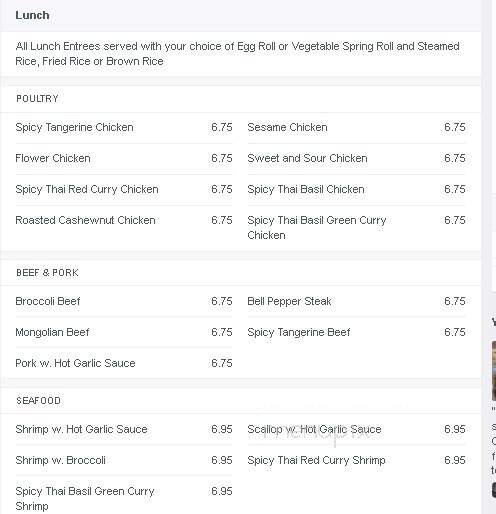This rectangular menu, oriented vertically, features a clean white background with predominantly black text. In the upper left corner, the menu is headed with the word "Lunch" in bold. Just below, a note informs patrons that all lunch entrees are served with a choice of an egg roll or a vegetable spring roll, along with steamed rice, fried rice, or brown rice. 

### Poultry
- Spicy Tangerine Chicken: $6.75
- Flour Chicken: $6.75
- Spicy Thai Red Curry Chicken: $6.75
- Roasted Cashew Nut Chicken: $6.75
- Sesame Chicken: $6.75
- Sweet and Sour Chicken: $6.75
- Spicy Thai Basil Chicken: $6.75
- Spicy Thai Basil Green Curry Chicken: $6.75

### Beef and Pork
- Broccoli Beef: $6.75
- Mongolian Beef: $6.75
- Pork with Hot Garlic Sauce: $6.75
- Bell Pepper Steak: $6.75
- Spicy Tangerine Beef: $6.75

### Seafood
- Shrimp with Hot Garlic Sauce: $6.95
- Shrimp with Broccoli: $6.95
- Spicy Thai Basil Green Curry Shrimp: $6.95
- Scallops with Hot Garlic Sauce: $6.95
- Spicy Thai Red Curry Shrimp: $6.95

Each section of the menu is clearly delineated by gray lines between items, with a prominent long gray line separating the header from the rest of the content, ensuring an organized and easy-to-read layout.